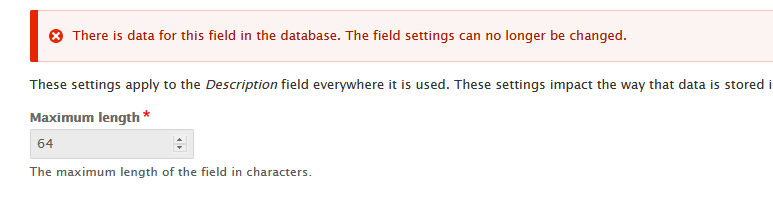A screenshot of a website interface is displayed, featuring a predominantly white background. At the very top, a solid red banner spans horizontally, with a red circle containing a pink X icon situated prominently within the banner. The text in the banner reads, "There Is Data For This Field In The Database. The Field Settings Can No Longer Be Changed." in a burgundy red font, with each word in the first sentence capitalized.

Beneath this banner, on the white background, black text states, "These settings apply to the Description field, everywhere it is used. These settings impact the way that data is stored." The word "Description" is capitalized and slightly italicized. 

Further down, bold black text with a red asterisk marks the label "Maximum Length," beginning with a capital M. Adjacent to this label, there is an input field set to '64' with up and down arrows for adjustment. The text below this states, "The maximum length of the field in characters."